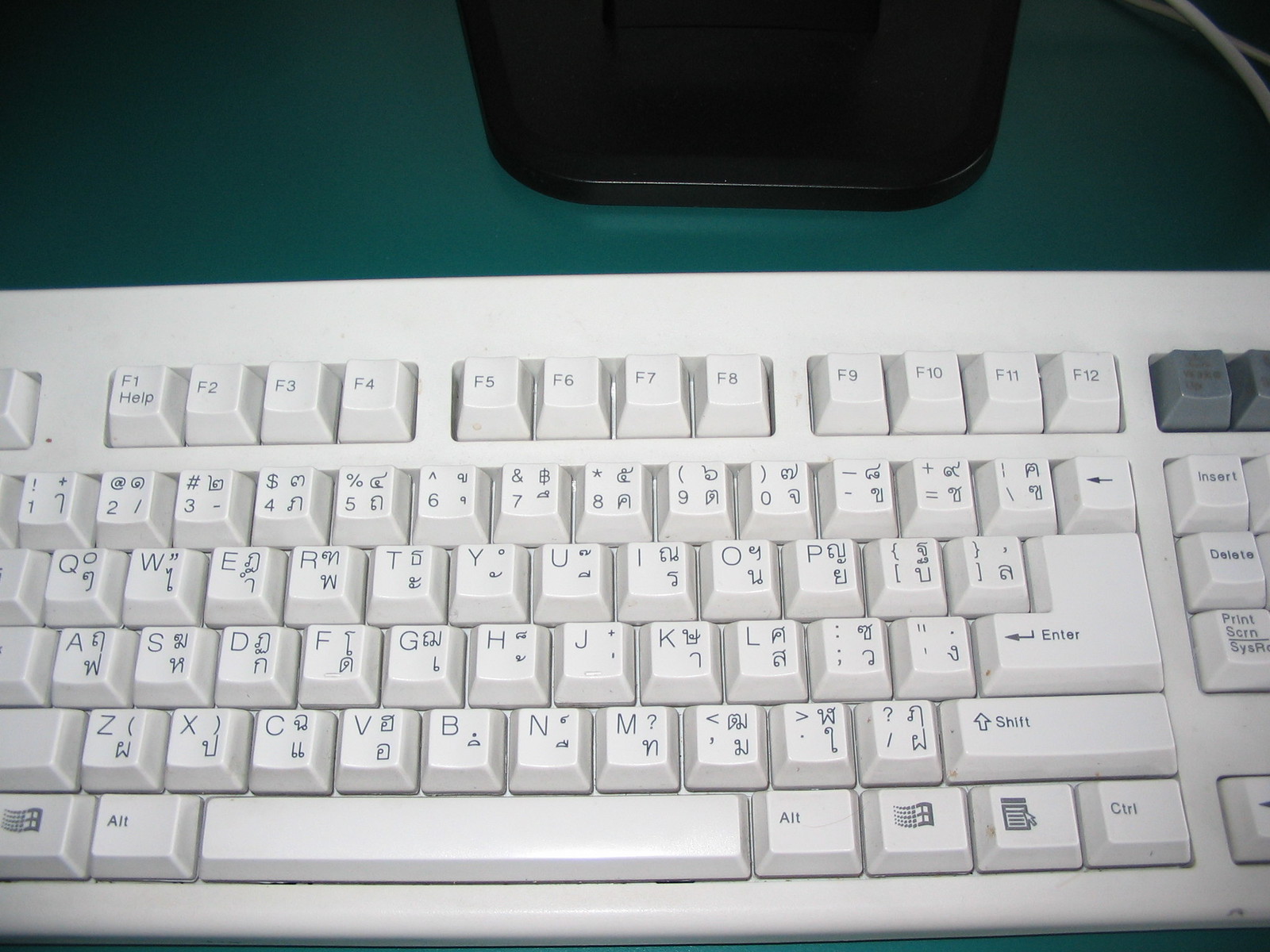The photo captures a top-down view of a slightly aged, off-white keyboard resting on a dark green desk. The keyboard features traditional English symbols along with unusual pictographic characters on each key, resembling intricate, non-Asian squiggles or potentially Egyptian-like symbols. The keyboard appears complete with all the standard keys, including the function keys (F1-F12) in a row at the top, numbers, letters, and various control keys such as spacebar, alt, ctrl, and shift. There are visible hints of wiring suggesting it is a wired keyboard. This keyboard, with its 3D push-button keypads, evokes an older PC or Mac style, further indicated by the presence of a Windows logo. The image is cut off at both edges leaving out the caps lock, tab, shift, and insert buttons. At the top of the image, the base of a black lamp is visible.